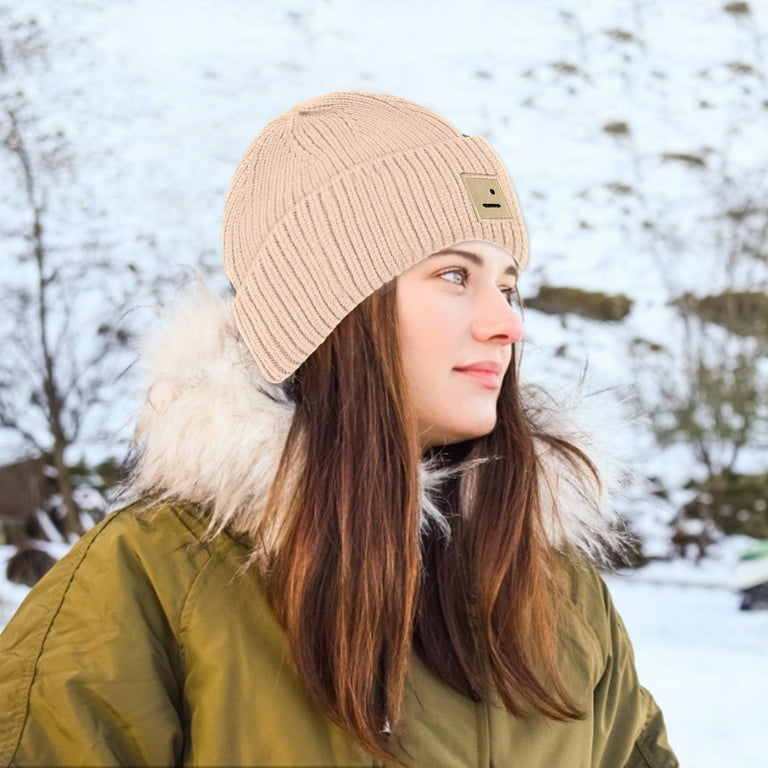The image depicts a close-up of a young woman with long brown hair, captured in a wintry scene. She is facing to the right and smiling slightly, her light-colored eyes and dark eyebrows adding to her cheerful demeanor. Her attire includes a green parka jacket with a white fur-lined hood that rests on her shoulders, and she sports a light pink knitted cap adorned with a small brown patch in the front. The background, which is out of focus, reveals snow-covered barren trees, further emphasizing the winter setting. The overall composition highlights the woman’s enjoyment of the snowy environment.